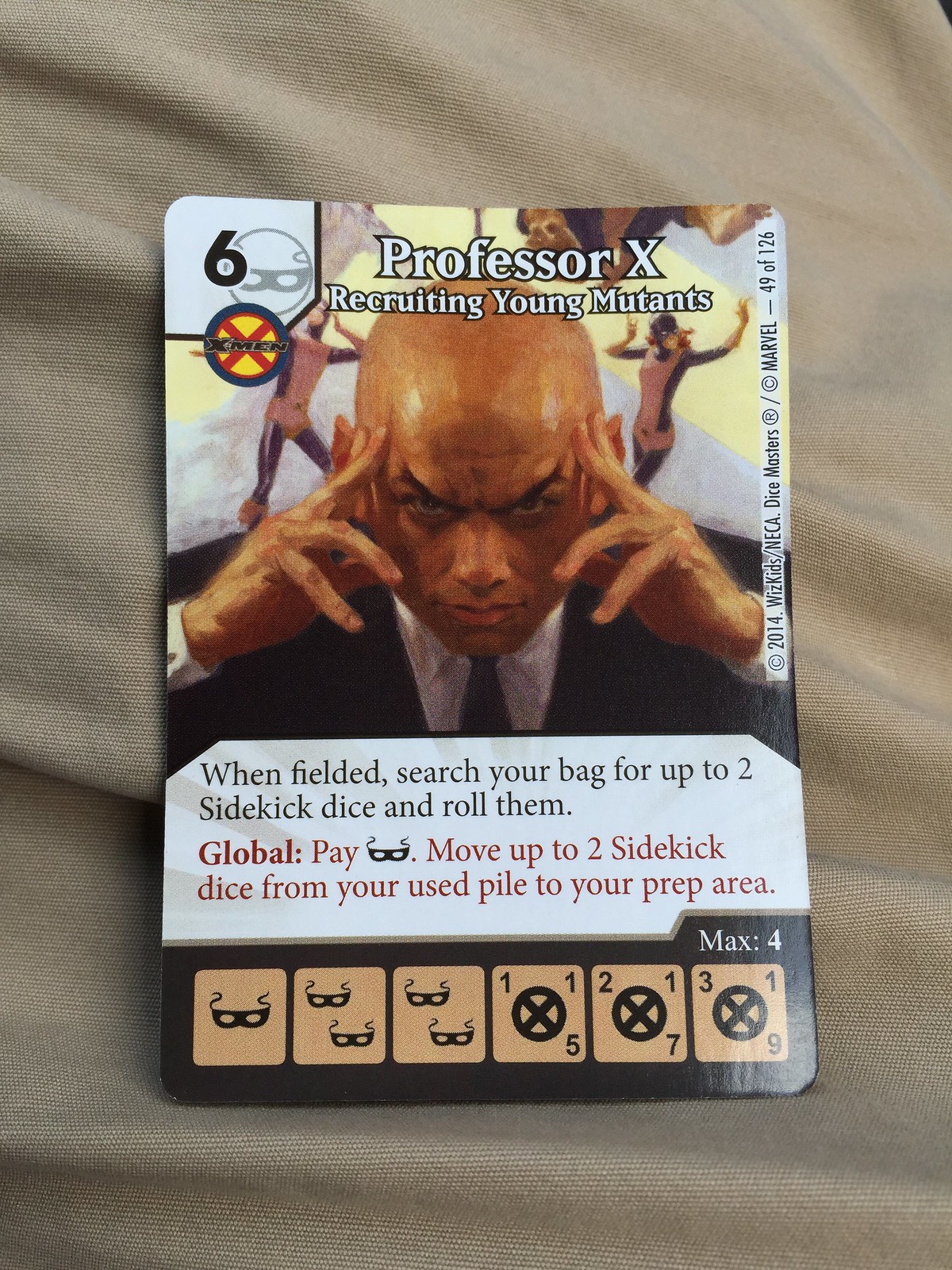The image depicts a collectible playing card from a game, set against a light brown fabric background, possibly a piece of clothing or a pillow. The card features a prominent black number "6" inside a white square in the upper left-hand corner, along with some emblematic icons nearby. At the top, in white text, it reads "Professor X" with the subtitle "Recruiting Young Mutants". The central image showcases a bald man, identified as Professor X, dressed in a suit and shown from chest up. He has thin eyebrows, a serious expression, and he is looking directly ahead with his fingertips pressed to his forehead. Behind him are costumed figures accentuating his focus. Below the image, there's a white text box that details the card's effects: "When fielded, search your bag for up to two sidekick dice and roll them." Additionally, in red text, it states: "Global Pay [mask icon]: Move up to two sidekick dice from your used pile to your prep area." The bottom of the card features six small boxes with various icons and numbers, providing further specific information, including symbols like masks and circles with X's inside them, along with numerical values indicating different attributes or abilities of the card.